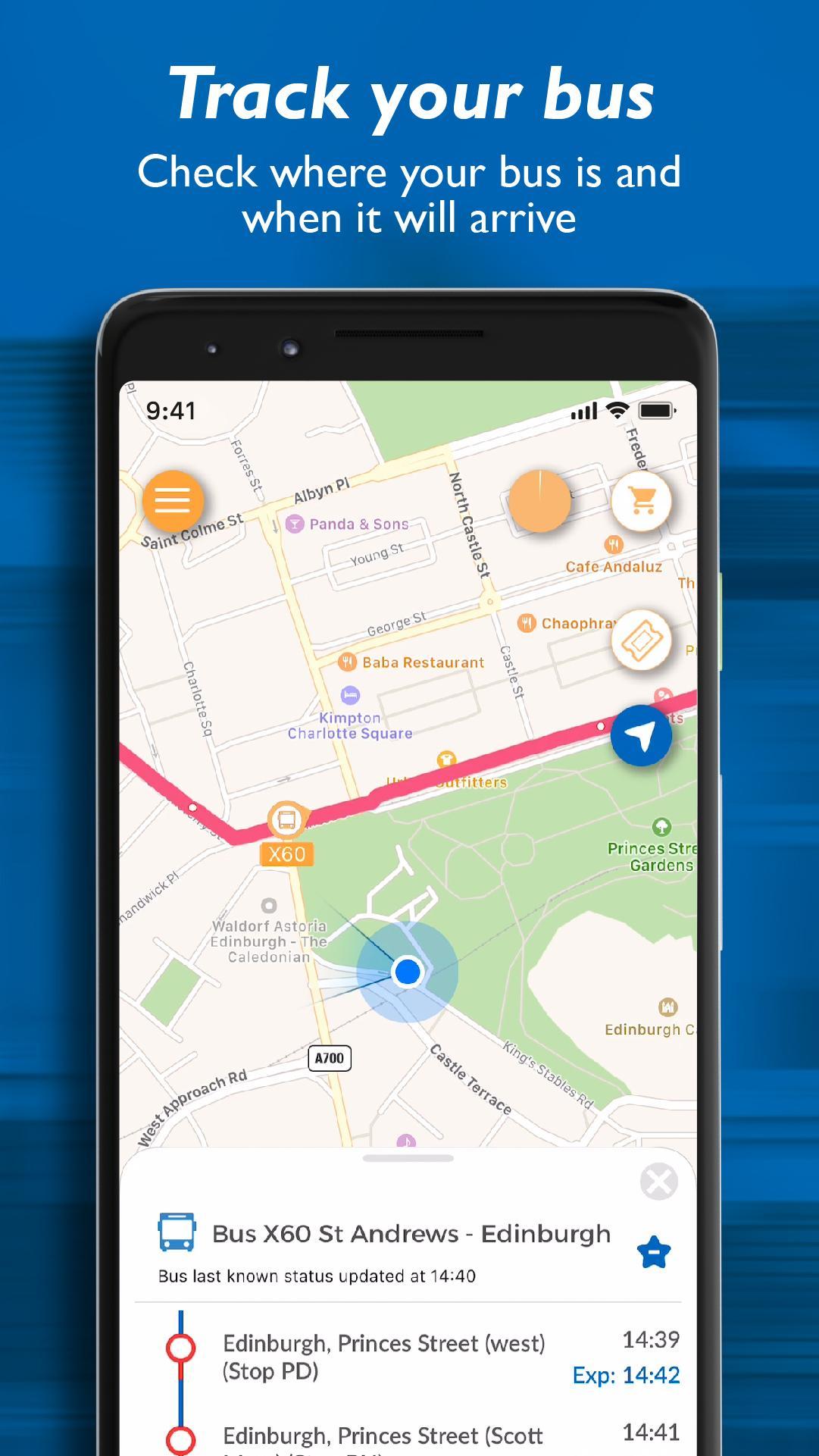This image features a blue background with a smartphone displaying a bus tracking application. Above the smartphone, white text reads: "Track your bus, check where your bus is and when it will arrive." The app interface on the smartphone screen showcases a map with a highlighted bus route in pink. A blue location pin marks the bus's position on the map.

Centered on the map is another blue dot and a text that reads: "Bus: X60, St Andrews, Edinburgh". The bus's last known status was updated at 14:40 at Edinburgh, Princess Street, West, stop PD, with the expected arrival time at 14:42. The next stop, Princess Street, Scott, is indicated with an arrival time of 14:41, which is also the bus's final destination.

An orange bus icon on the map is labeled "X60," which corresponds to the bus number. The app is designed to help users track the real-time location and status of their bus along its route, ensuring they are informed of where the bus is and when it will arrive. The bus's route is clearly marked in pink, navigating past the Kimpton Charlotte Square in Edinburgh.